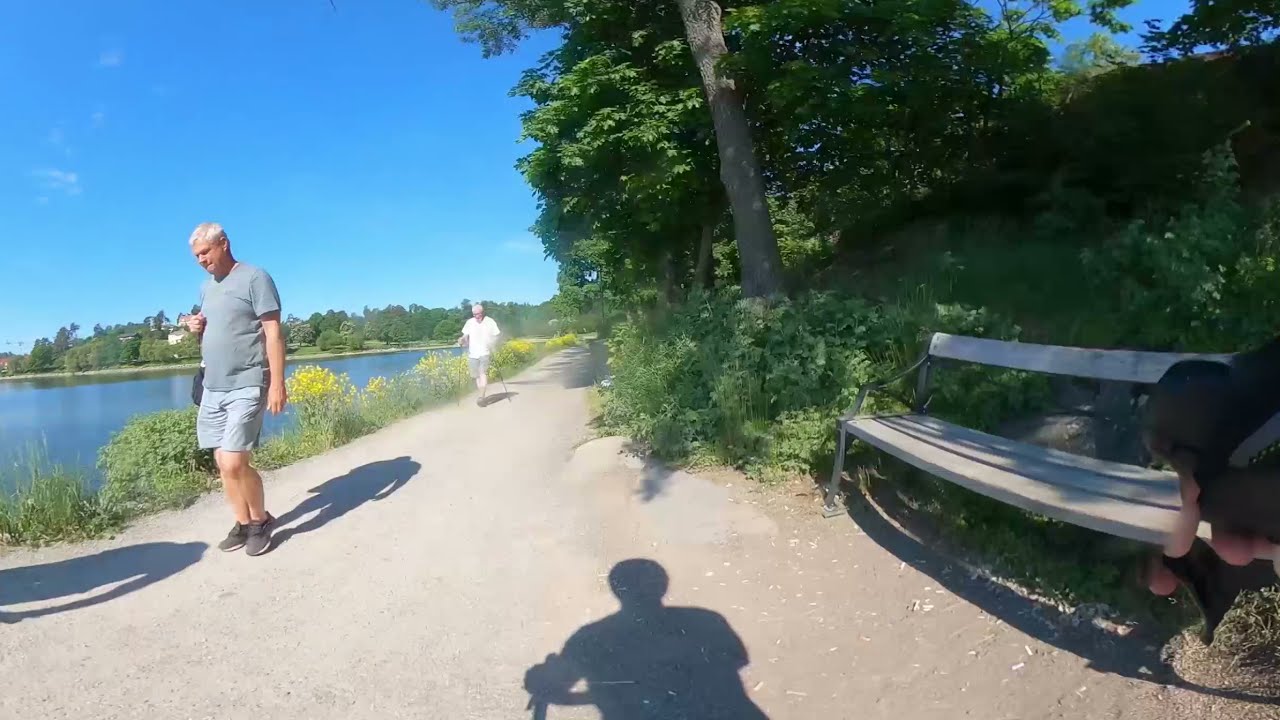The image showcases a serene outdoor scene set in a public park during the middle of the day. Dominating the center of the picture is a dirt-and-gravel walking path where two men are walking towards the camera. The man in the foreground wears a blue T-shirt, grayish-blue shorts, and dark shoes, while behind him, another man is donned in a white shirt and light blue shorts. Both have silver hair. A shadow of a bicyclist, moving in the opposite direction of the walking men, stretches across the path.

To the left of the path lies a tranquil lake, bordered by a variety of green and yellow shrubs. Further back, across the lake, a row of trees can be seen, enhancing the natural atmosphere of the scene. On the right side of the image, there's a slightly grassy slope ascending into an area filled with wild bushes and trees. A park bench is situated near the bottom right corner of the image, with someone seated and obscured by foliage. The sky above is predominantly blue with a few scattered clouds, providing a bright and pleasant backdrop to this picturesque park setting. The colors in the image include shades of blue, white, gray, green, yellow, and tan. The overall composition, with the walking path at its center, vividly captures the peacefulness and natural beauty of an outdoor park environment.